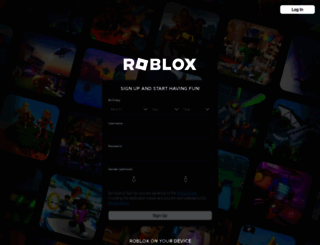In the center of this small image, the word "Roblox" is prominently displayed at the top in white text, with the first "O" stylized as a slightly tilted square. Beneath this, a dialogue box with a black background contains white text instructing users to "Sign up and start having fun." Below this prompt, there is a field labeled "Birthday," followed by input boxes for the day, month, and year of birth. The next field, "Username," features an empty input box underneath, and directly below it is the "Password" field with its corresponding input box.

Following these, there is a field for "Gender (optional)" which includes selectable icons for male and female. Beneath these options, there is some white blurry text alongside three green hyperlinked text elements. At the bottom of the dialogue box, a white "Sign Up" button with black text invites users to complete the registration. At the top right corner of the image is a "Login" button, which is also white with black text.

The background of the image features a colorful array of approximately 20 game screenshots, each contained within its own box and arranged at varying angles, giving a dynamic and vibrant feel to the overall image.